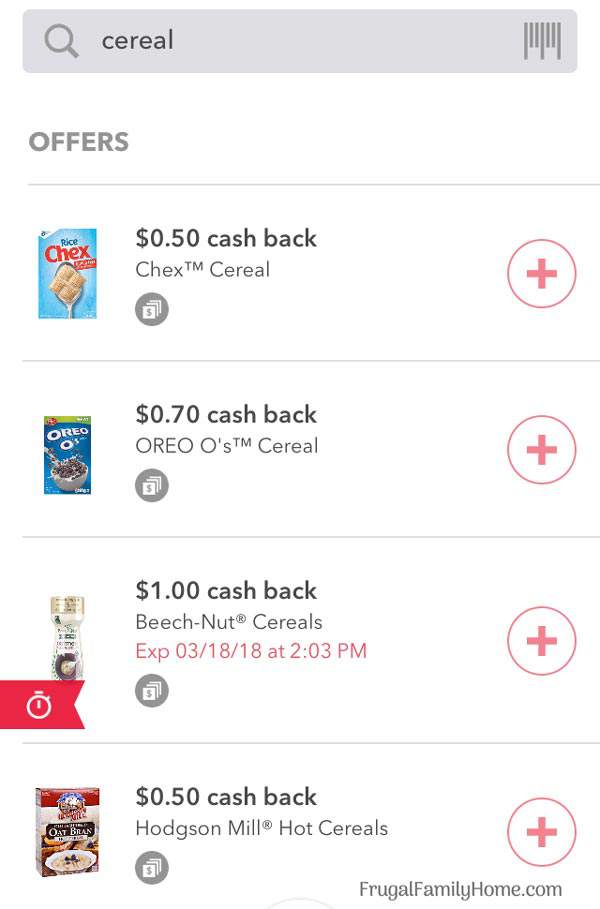A screenshot of the Frugal Family Home website displayed on a mobile phone, showcasing a search for "serial" in the search bar at the top. The screen presents a list of coupon offers under the heading "offers". Each listed item features a thumbnail image of the cereal box or package on the left, followed by the coupon title detailing the discount and the brand name. For example, the first item displays a Rice Chex box with a coupon title stating "50 cents cash back Chex cereal." On the far right of each item, there's a prominent red circle with a white plus sign, indicating an option to add the coupon to the user's account. The website’s name, frugalfamilyhome.com, is visible at the bottom of the screen, confirming the source of the screenshot.